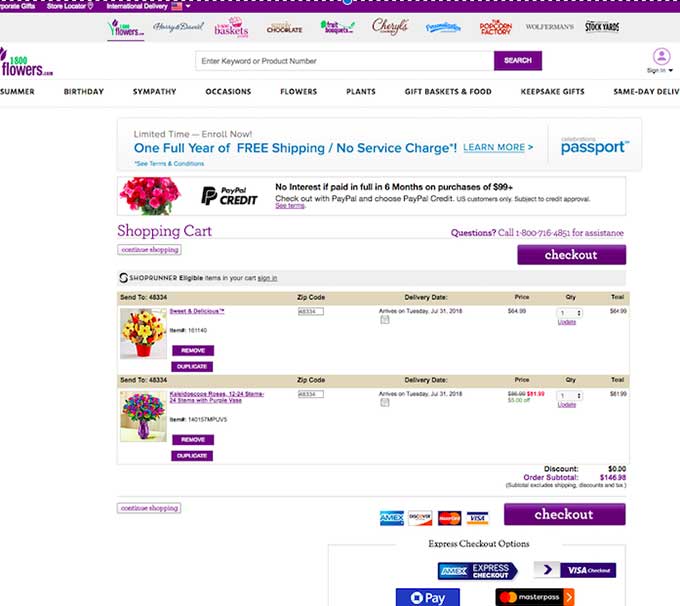Displaying the homepage of 1800flowers.com, this image showcases the website's primary features and navigation elements, albeit with some blurriness. The purple banner at the top, partially visible, highlights the international delivery service, with the American flag selected as the current locale. Beneath the banner, a series of logos represent affiliated brands including 1-800-Flowers, Cheryl's Cookies, The Popcorn Factory, Stockyards, and more.

The upper-central section features a search bar inviting users to enter keywords or product numbers, alongside a sign-in option. Below, bold black lettering directs visitors to various categories such as Birthday, Sympathy, Occasions, Flowers, Plants, Gift Baskets & Food, Keepsake Gifts, and Same Day Delivery.

The focal point of the image appears to be the user's shopping cart, containing two bundles of flowers with a subtotal of $146.38. Checkout options and payment methods, including American Express, MasterCard, and Visa, are visible at the bottom, indicating the final steps of the purchasing process.